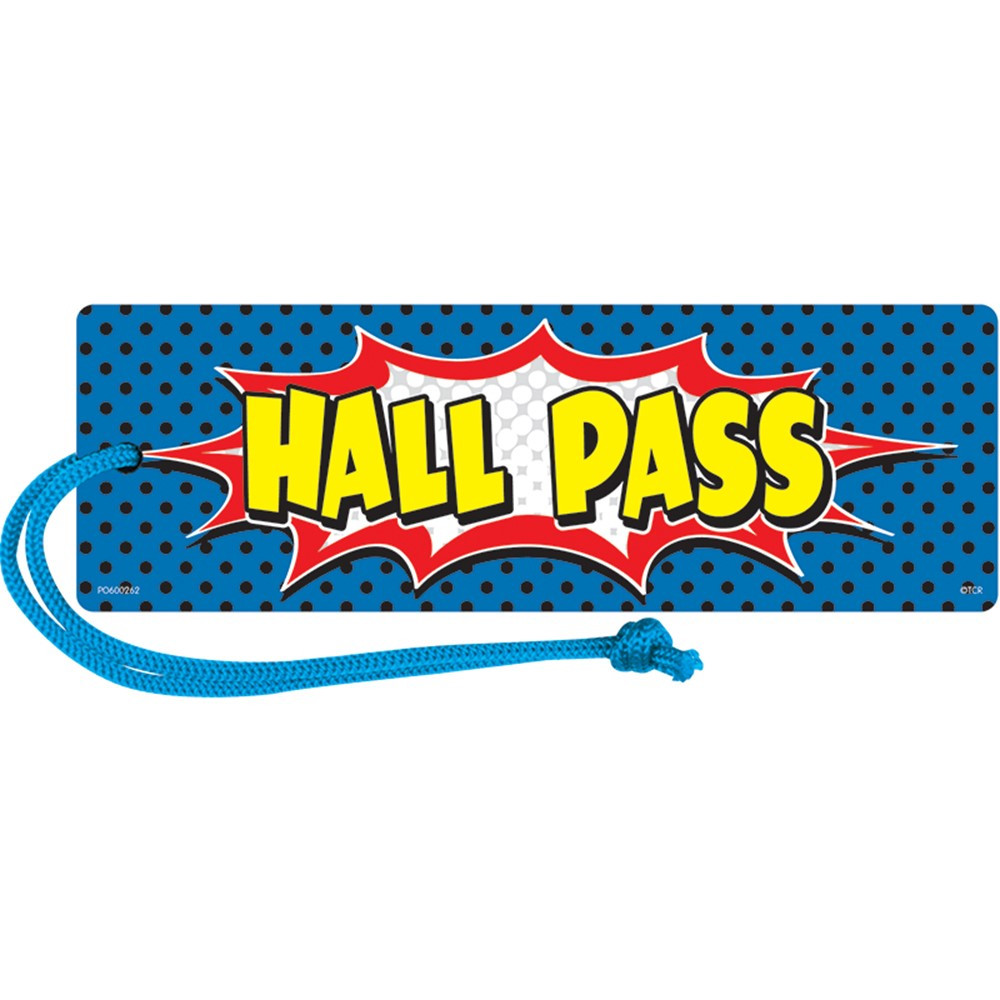The image depicts a rectangular, blue plastic Hall Pass, embellished with uniform black polka dots. The Hall Pass is wider than it is tall and has a hole on the left side through which a blue rope, reminiscent of a shoestring, is threaded, allowing it to be worn around the neck or wrist. The pass features the words "Hall Pass" prominently in the center, presented in stark yellow, cartoonish letters with a black border and shadowing. Behind these letters, there’s an explosion emblem similar to the "kapow" or "bam" visuals from children’s television shows. This emblem comprises a red border with a smaller white border inside, surrounding a translucent center containing gray and white patterns that create a dynamic, almost fiery effect against the blue and black polka-dotted background.